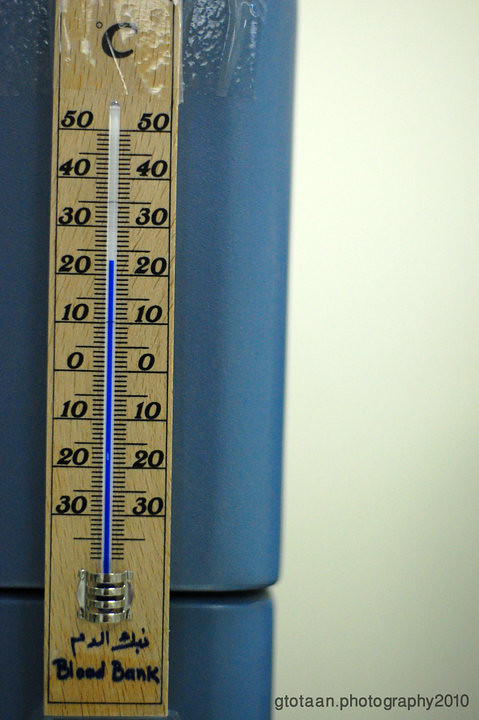A close-up image captures a wooden-framed wall thermometer affixed to the blue door of a refrigerator using clear transparent tape. The thermometer, designed for Celsius measurements, prominently displays a large black "C" at its top. It features a wide-ranging scale that spans from -30 to 50 degrees Celsius. The blue liquid indicator currently marks the temperature at 23 degrees Celsius. Notably, the base of the thermometer bears the inscription "Blood Bank" in bold black ink, indicating its specific usage for monitoring temperature in such environments.